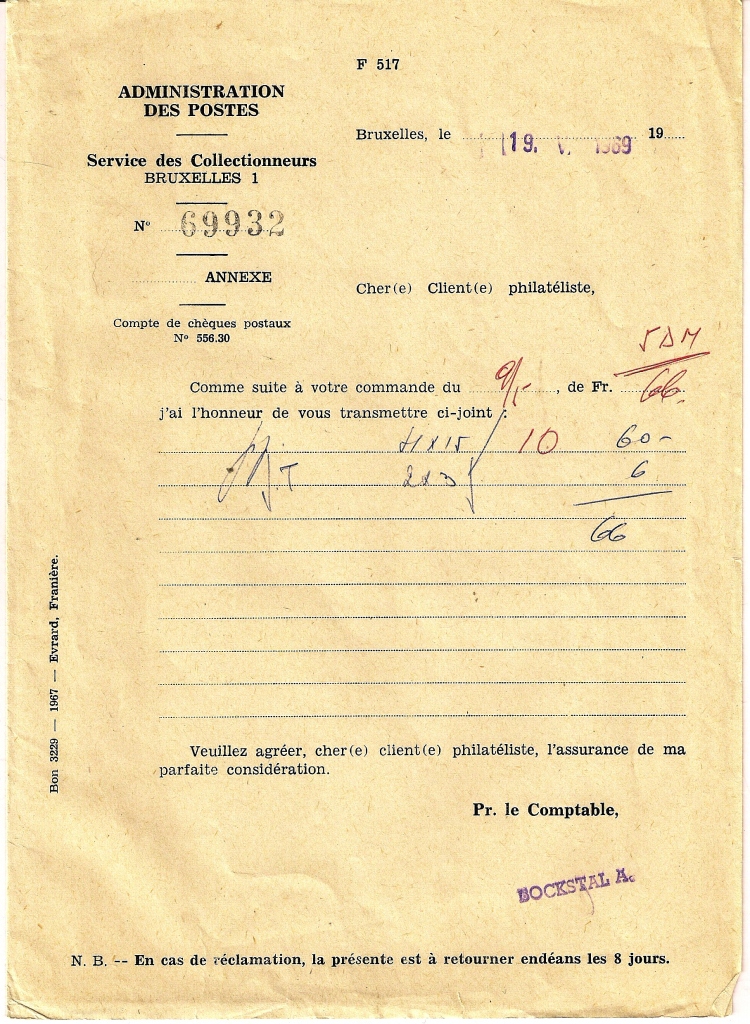This image depicts a weathered, yellowed receipt, predominantly typed in French. The paper, dating back to 1969, shows clear signs of age with noticeable creases and folds. The header reads "administration de posts" in French, reflecting its non-English origin. The main body consists of typed text interspersed with handwritten numbers, some in red and others in blue ink, suggesting calculations such as "60 plus 6 equals 66". A prominent ink stamp bearing the number 69932 is visible, along with a purple date stamp. In the bottom right corner of the receipt, there's a stamp that reads "Boxtel A.".